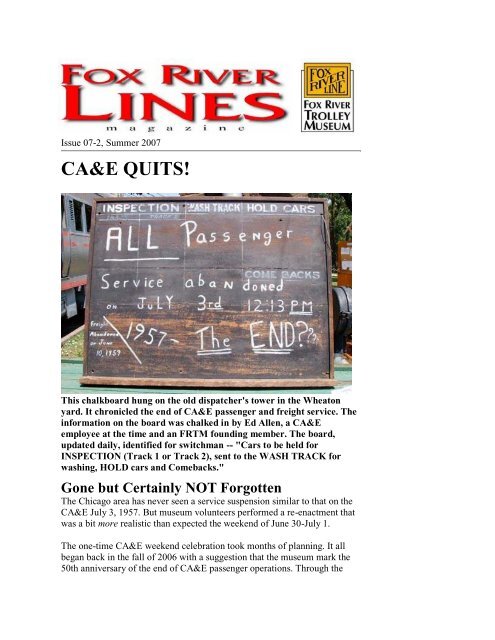This image appears to be the cover of the Fox River Lines Magazine, Issue 07-2, Summer 2007. The top of the page features the title "Fox River Lines" in bold red text, followed by the word "Magazine" in smaller text beneath it. On the right side, it indicates that the magazine is from the Fox River Trolley Museum. The cover prominently displays the headline "CA&E Quits!" in bold letters. Below this headline, there is a photograph of a chalkboard which reads, "Inspection, track, hold cars, all passenger service abandoned on July 3rd, 12:13 p.m., 1957 to the end?" This chalkboard, used by the CA&E employee Ed Allen, was hung on the old dispatcher's tower in the Wheaton Yard and marks the end of the Chicago, Aurora, and Elgin Railroad’s passenger and freight service, as chronicled by Allen, who was also a founding member of the Fox River Trolley Museum.